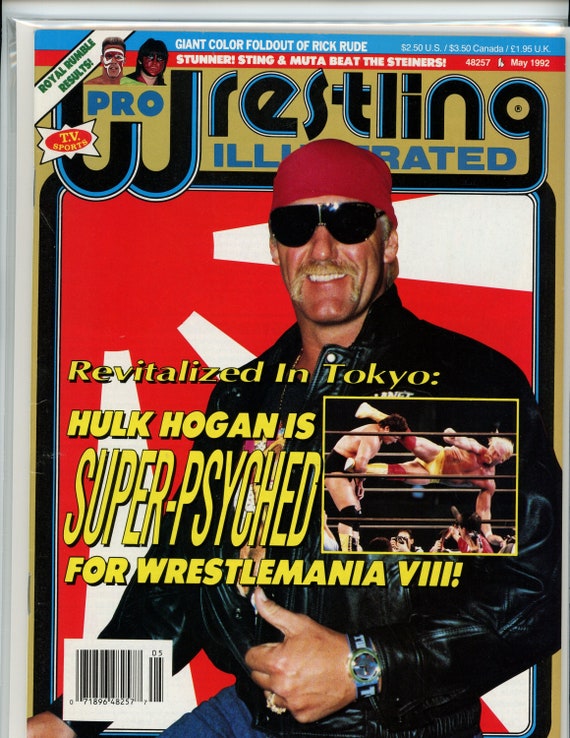This full-color, vertically rectangular cover of "Pro Wrestling Illustrated," from May 1992 and priced at $2.50 in the U.S., features a vibrant design with an off-white border. Dominating the cover is a large image of Hulk Hogan. He sports a red bandana, sunglasses, and a black leather jacket over jeans, revealing his signature blonde mustache. Hogan is captured smiling at the camera while giving a thumbs up with his left hand. Overlaying this image is a bold headline in gold that reads, "Revitalized in Tokyo: Hulk Hogan is Super Psyched for WrestleMania 8."

Additionally, the cover includes a smaller inset image of Hogan in his wrestling gear, delivering a kick to an opponent in the ring, possibly Andre the Giant. Above the main image, the magazine title, "Pro Wrestling Illustrated," stands out in a blue and red header. The cover also features a banner that highlights "Royal Rumble Results" and mentions a "Giant Color Foldout of Rick Rude."